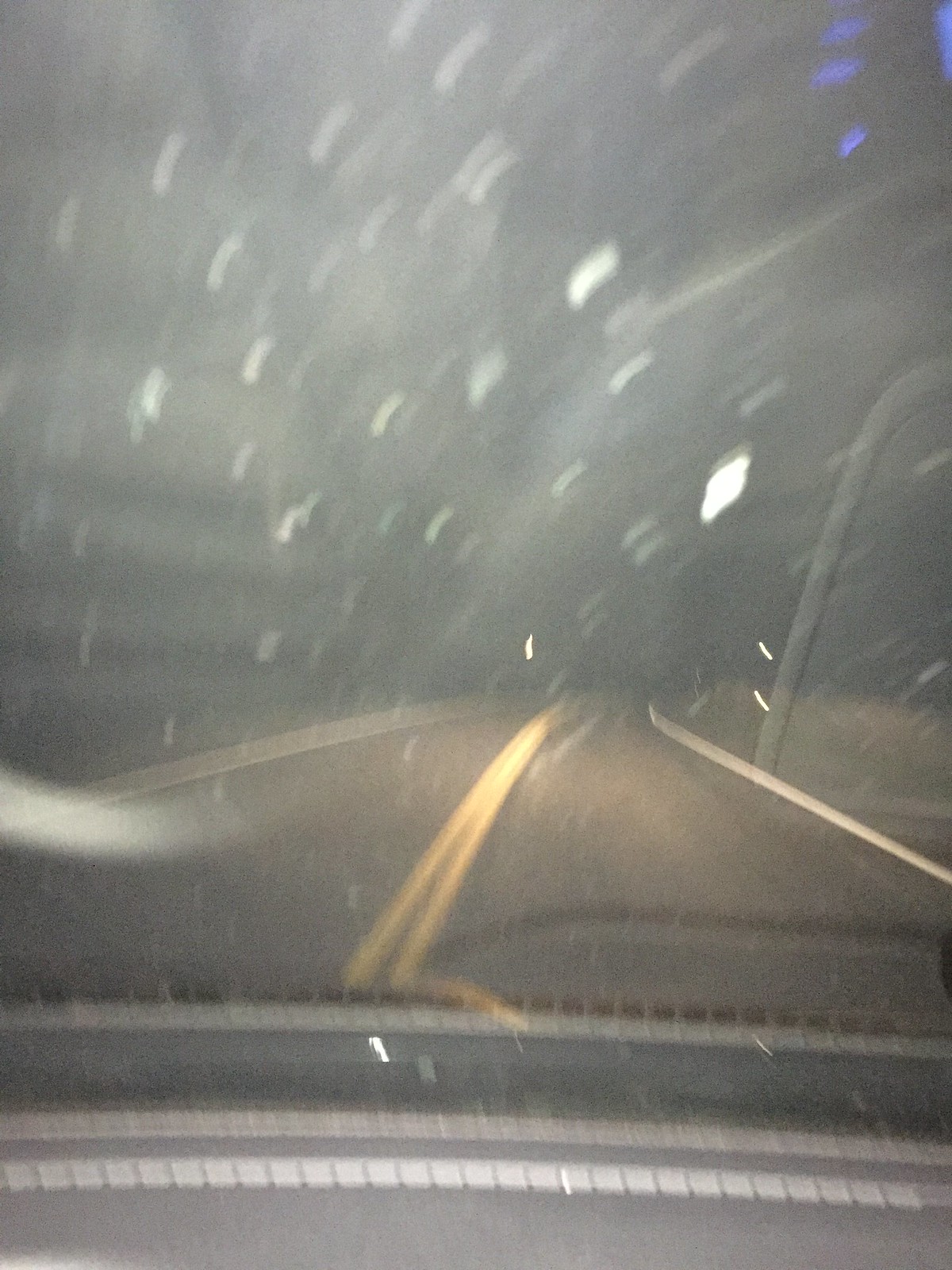A blurry nighttime photograph taken from inside a car, likely from the passenger's seat but slightly centered, captures a wintry scene through the windshield. The image, approximately 50% taller than it is wide, reveals a gray dashboard spanning the bottom of the frame. Outside, the road ahead, illuminated by headlights, shows two defined lanes with double yellow lines in the center and white lines marking the road's edges. The road curves slightly to the right. Thick snowflakes are visibly falling, adding a stormy atmosphere to the black, cloud-streaked sky. The car’s motion and dark surroundings make details beyond the road difficult to discern. Reflective elements in the windshield and a faint interior light create a sense of being in motion on a snowy night.